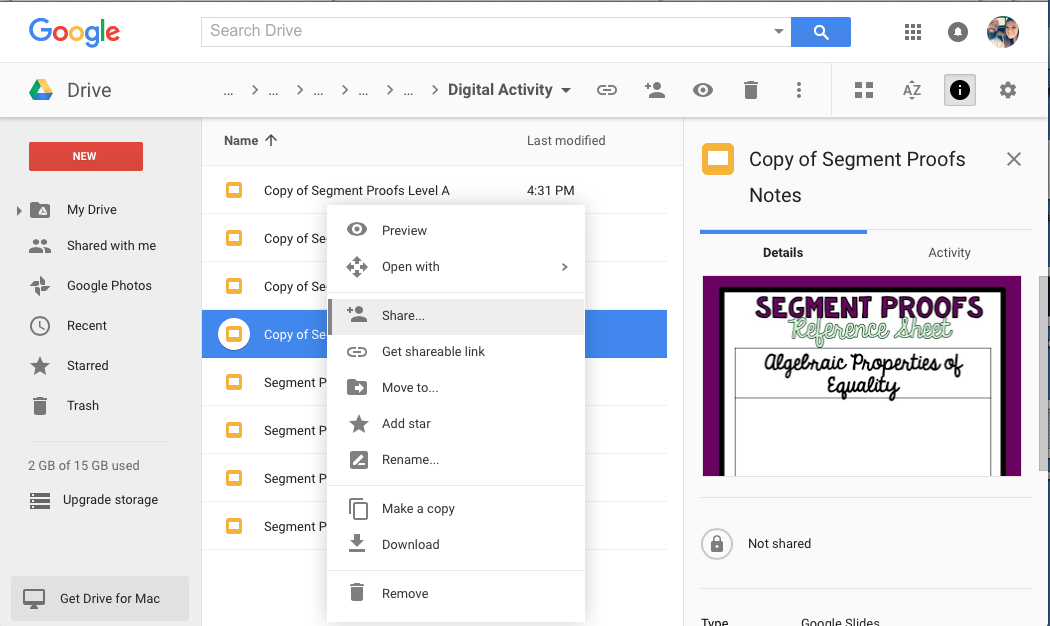This image captures a detailed view of Google's homepage, specifically focusing on the Google Drive interface. The layout is framed by a thin black border along the top and right side, with a white margin about an inch from the top. In the upper left corner, prominently displayed, is the iconic "Google" logo. Approximately an inch to the right of the logo, there is a search bar extending horizontally.

An inch from the right edge, text in black reads "Search Drive." Adjacent to this, on the right, is a blue tab featuring a white search icon. Below it, three rows of three black dots are aligned. A black circle encompasses a white bell icon beside a profile picture depicting a bearded man on the left and a woman on the right, visible only by their heads.

To the left, occupying about an inch, there is a light gray section. Within this space, a tri-colored triangle appears with a blue base, yellow side, and green bottom. Adjacent to it, the word "Drive" is displayed in black. Below "Drive," a series of dropdown tabs spans the width of the section.

Under the "Drive" title, a light blue border extends for about two inches across the top. A red tab labeled "New" in white text sits at the top of this section. Beneath it, six tabs are available for interaction, each marked by black lettering alongside icons. Below this setup, a storage usage indicator reads "2.2 GB of 15 GB used," with an "Upgrade storage" option next to it, marked by three horizontal lines.

Towards the right, the word "Name" is followed by eight clickable options, the fourth highlighted by a blue rectangle. An information pop-up overlays this section. Additionally, a small yellow square containing a white segment is labeled "Copy of Segment Proofs," followed by sections for "Notes" and "Detail activity" with further information underneath.